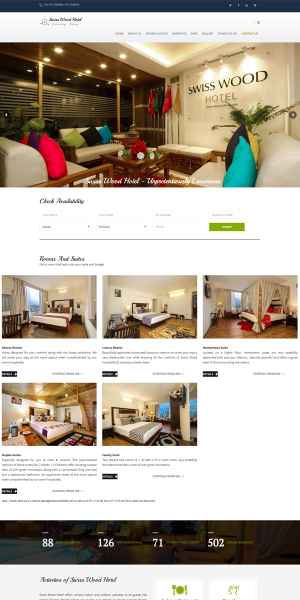The image depicts a webpage from a hotel website called "Swiss Wood Hotel." The top part of the page features a prominent blue bar that includes a contact phone number and various social media links. The navigation menu offers several tabs such as "Home" and "About Us," with one tab highlighted in green, displaying the website name in a black cursive font. 

Beneath the navigation bar, there's a large image of the hotel's lobby, showcasing an elegant seating area with wooden tables and a selection of international flags. Adjacent to this image is a "Check Availability" section, which provides various options and input boxes for prospective guests. 

Further down, the webpage displays five room listings, each accompanied by an image of the room. These rooms feature hardwood flooring, a range of bed sizes, and various amenities depending on the room type. 

Towards the bottom, the page lists several contact numbers in white text and highlights that the hotel includes a restaurant and diverse food offerings. The overall page design maintains a clean look with a primarily white background.